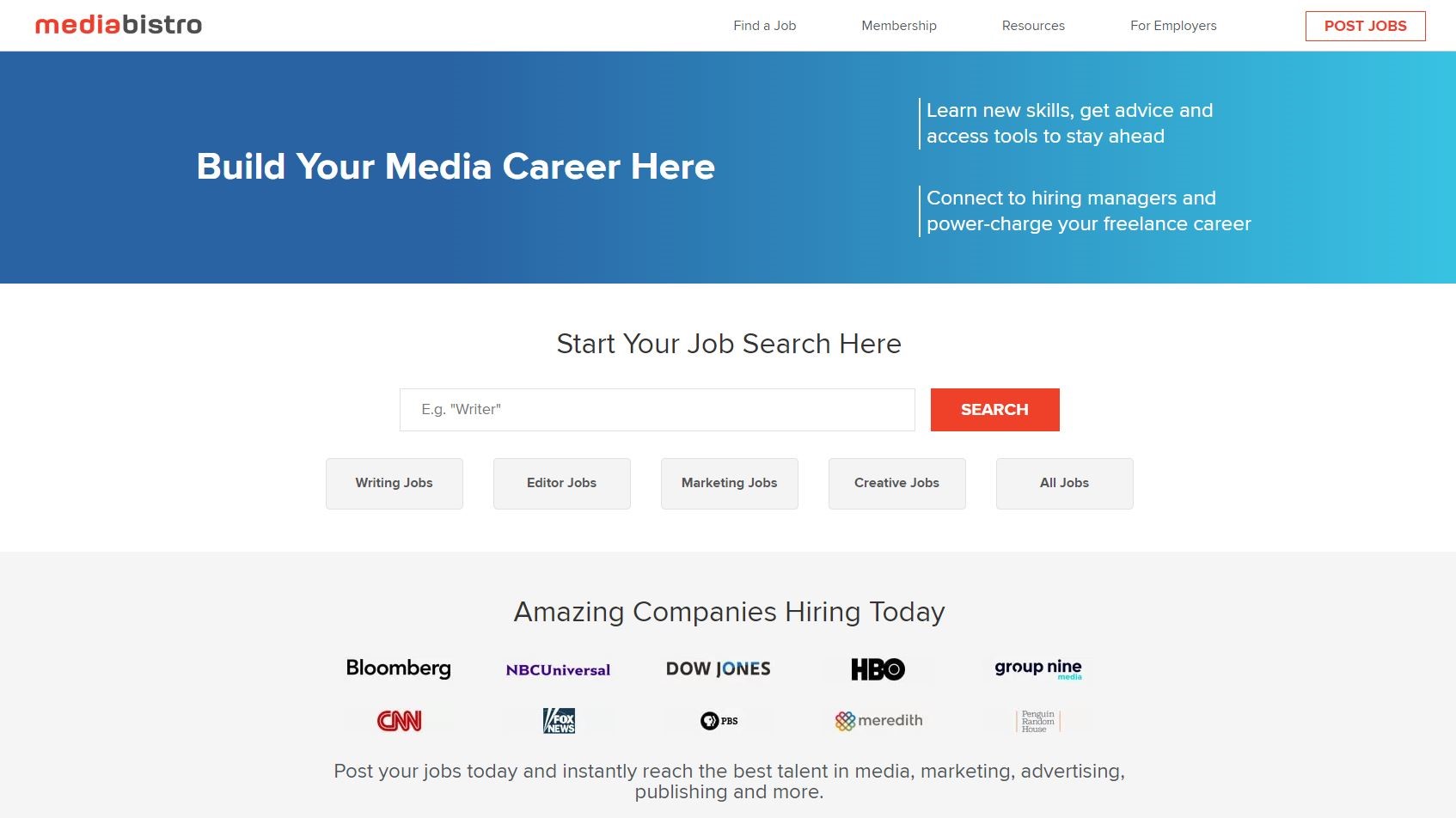Screenshot of a website named Media Bistro, showcasing a clean and professional design.

The layout features a primarily white background for the main body. Across the top is a prominent blue banner, which transitions from dark blue on the left to light blue on the right, complemented by a white navigation bar above it. The top left corner displays the Media Bistro logo in all lowercase letters, with "media" in red and "bistro" in black.

Centered in the white navigation bar are various options:
- Find a Job
- Membership
- Resources for Employers

In the top right corner is a conspicuous white button with a red outline, marked "Post Jobs" in red text.

The blue banner below the navigation bar prominently displays, in large white font on the left side: "Build Your Media Career Here." On the right side, transitioning to light blue, additional motivating text reads:
"Learn new skills, get advice, and access tools to stay ahead.
Connect to hiring managers and power-charge your freelance career."

Beneath the blue banner, centrally located, is an inviting section labeled "Start Your Job Search Here," followed by a search bar. To the right of the search bar is an orange button with "Search" written in white.

Below the search bar are categories for job searches:
- Writing Jobs
- Editor Jobs
- Marketing Jobs
- Creative Jobs
- All Jobs

A pale gray banner beneath these job categories showcases companies currently hiring, with logos for:
- Bloomberg
- HPC
- Universal
- Dow Jones
- HBO
- Group 9
- CNN
- Meredith
- Two additional logos that are too small to read.

The page concludes with a call-to-action: "Post your jobs today and instantly reach the best talent in media, marketing, advertising, publishing, and more."